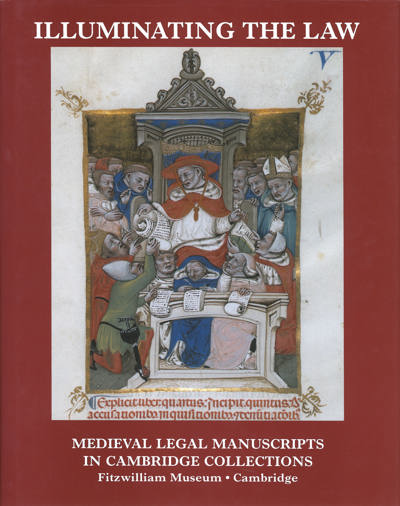The image depicts what appears to be a book cover with a rectangular shape. The outer frame of the cover is maroon, and within it is a white panel featuring a detailed and ornate medieval scene. At the top of this panel, the title "Illuminating the Law" is prominently displayed in white text. Below the title, there is an inscription that reads "Medieval Legal Manuscripts in Cambridge Collections, Fitzwilliam Museum, Cambridge."

Central to the illustration is a man seated on a very ornate throne, surrounded by around a dozen figures. The man, adorned in a white robe with red accents and a red hat, appears to be an authoritative figure. He holds a parchment in his left hand and seems to be receiving another document from a person to his right. The background behind him is gold, enhancing the regality of the scene.

The figures surrounding him, some bearing scrolls and books, look towards him, seemingly seeking guidance or delivering messages. Among the gathered individuals, one is particularly notable for wearing what resembles a Pope's hat. The scene is vividly colored, with shades of black, white, gray, gold, red, blue, and green.

Below the central illustration, there is some text written in red, though its language is not identifiable. The painting on the cover looks professionally executed, possibly indicating it was reproduced from an original medieval manuscript.